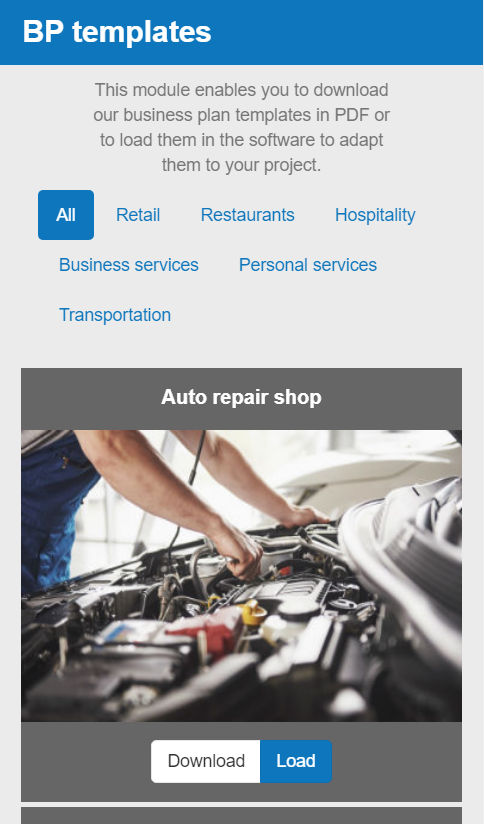The screenshot features a vertically-oriented rectangle, approximately twice as tall as it is wide. At the very top, it displays a blue header with the text "BP Templates" in a white font, where "BP" is capitalized and "Templates" is in lowercase.

Below this header lies the top half of the image with a light gray background containing a slightly darker gray text that reads: "This module enables you to download our business plan templates in PDF or to load them in the software to adapt them to your project."

Further down, there is a navigation menu. On the left side of the menu is a blue square with the word "All" written in white. Adjacent to this are several other categories written in blue, presumed to be hyperlinks: Retail, Restaurants, Hospitality, Business Services, Personal Services, and Transportation.

The bottom half of the image showcases a photo of the interior of a vehicle's hood. Visible in the photo are the forearms of a man with pale skin, and the left side of his torso, which is partially clad in a blue shirt. Directly above the photo, a gray border contains the white-font text "Auto Repair Shop." At the bottom of the image, another gray border presents two buttons: a white rectangle with "Download" written in gray font, and next to it, a shorter rectangle with "Load" in white font.